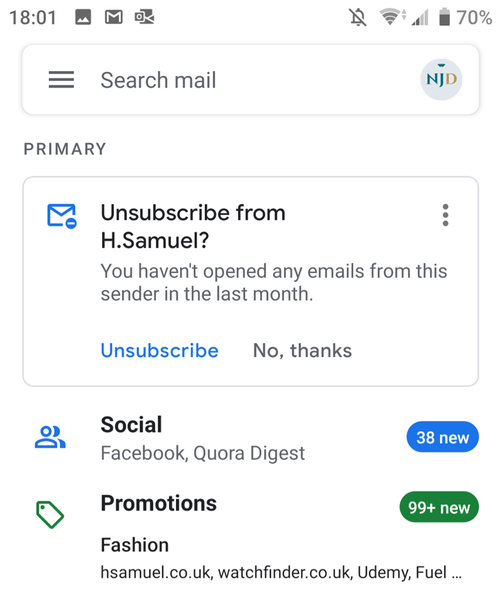This image features the screen of a cell phone displaying the main interface of someone's Google Mail account. In the top left corner, the time is indicated as 18:01 alongside the Google Mail icon. The top right corner shows a set of icons including a muted bell, wireless connection, cellular connection, and a battery symbol indicating 70% charge.

Just below these icons is a search bar labeled "Search Mail." Beneath the search bar, the word "Primary" signifies the primary inbox, accompanied by an envelope icon. It indicates an email from H. Samuel with a subscription prompt, stating "Subscribe from H. Samuel." The email indicates that no mails from this sender have been opened in the last month. Two options follow this prompt: "Unsubscribe" in blue text and "No Thanks" in black text.

Directly below this section, on the left, we see the "Social" category, symbolized by an icon of two people, listing "Facebook" and "Quora Digest" as sources. To its right, a button with a blue background and white text announces "38 New" unread emails. 

Further down, the "Promotions" category is marked with a price tag icon and lists "Fashion," "hsamuel.co.uk," "watchfinder.co.uk," and "udemyfuel." Adjacent to this section is a green button with the text "99 Plus New" in white, signaling a high volume of new promotional emails.

The overall page design features a clean, white background, and there are no additional photos or decorative images present on the screen.